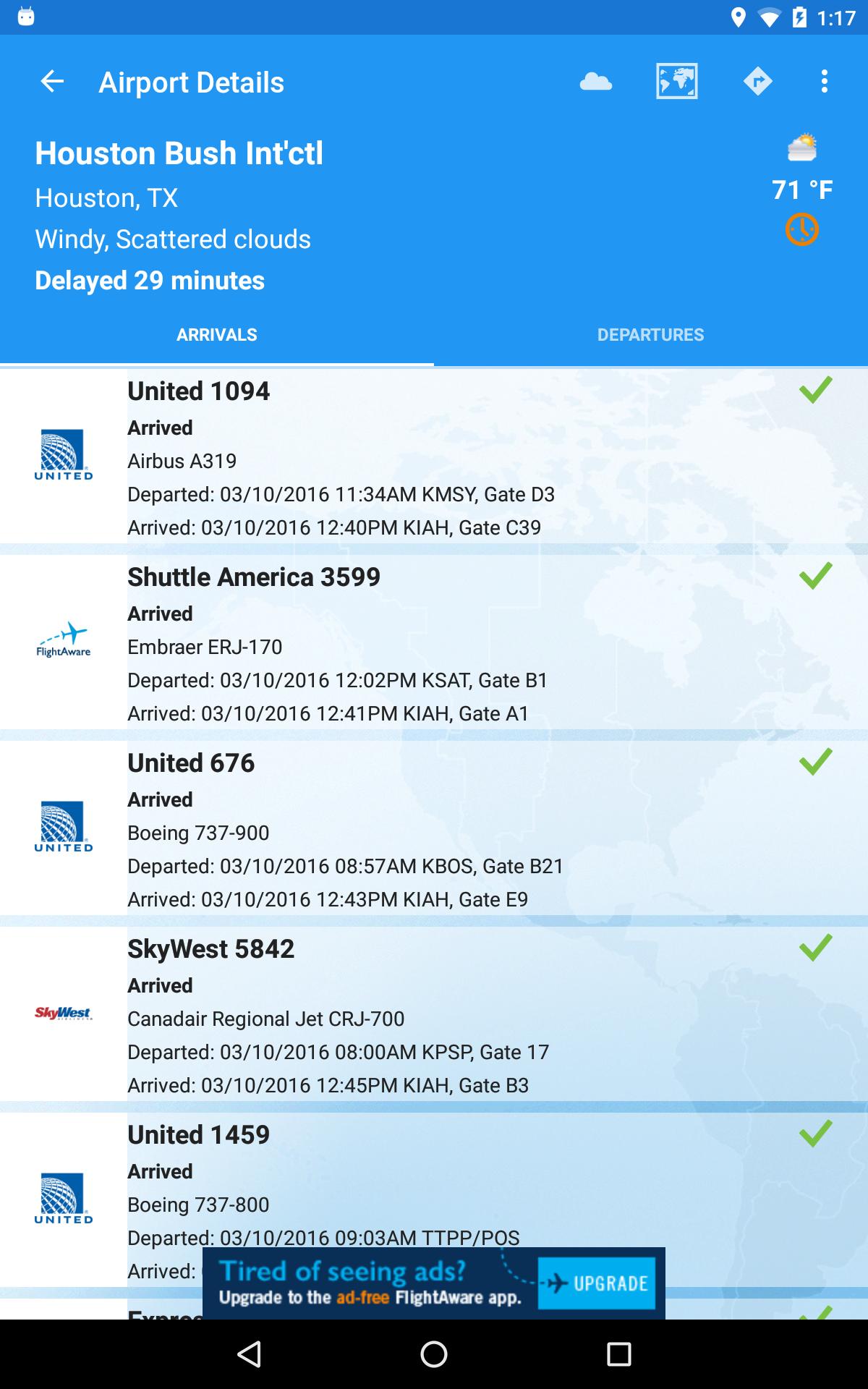The image displays a smartphone screen displaying a flight tracking application. At the top, the status bar shows icons for the time, battery, Wi-Fi signal, and location services. The upper portion of the screen has a blue header with white text that reads "Report Details." Below this header, the screen lists various flight information, denoted by their respective details and statuses.

The information encompasses flights arriving at Houston George Bush Intercontinental Airport (IAH), with current weather conditions described as windy with scattered clouds and a temperature of 71 degrees Fahrenheit. The interface features two tabs—"Arrivals" and "Departures"—with the "Arrivals" tab selected.

Detailed below are arrivals for the date, presumably October 10, 2016:

1. **United Flight 1094**:
   - Aircraft: Airbus A319
   - Departure: 10:34 AM from Louis Armstrong New Orleans International Airport (KMSY), Gate C3
   - Arrival: 12:00 PM at George Bush Intercontinental Airport (IAH), Gate C39

2. **Shuttle America Flight 3599**:
   - Aircraft: Embraer
   - Departure: 8:00 AM from an unspecified location
   - Arrival: 12:45 PM at George Bush Intercontinental Airport (IAH)

3. **United Flight 676**:
   - Aircraft: Boeing 737-900
   - Departure: 8:57 AM
   - Arrival: 12:43 PM at George Bush Intercontinental Airport (IAH)

4. **SkyWest Flight 5842**:
   - Aircraft: Canadair Regional Jet
   - Departure: 8:00 AM from an unspecified location
   - Arrival: 12:45 PM at George Bush Intercontinental Airport (IAH)

5. **United Flight 1459**:
   - Aircraft: Boeing 737-800
   - Departure: Data hidden
   - Arrival: Data hidden

At the bottom, there is a dark blue banner promoting an ad-free version of the app, which reads "Upgrade to the ad-free FlightAware app" with a blue upgrade button. The banner's text is a combination of blue, heart emoji, and orange font colors.

This image offers a comprehensive snapshot of flight arrival statuses, providing essential information for tracking and updates.